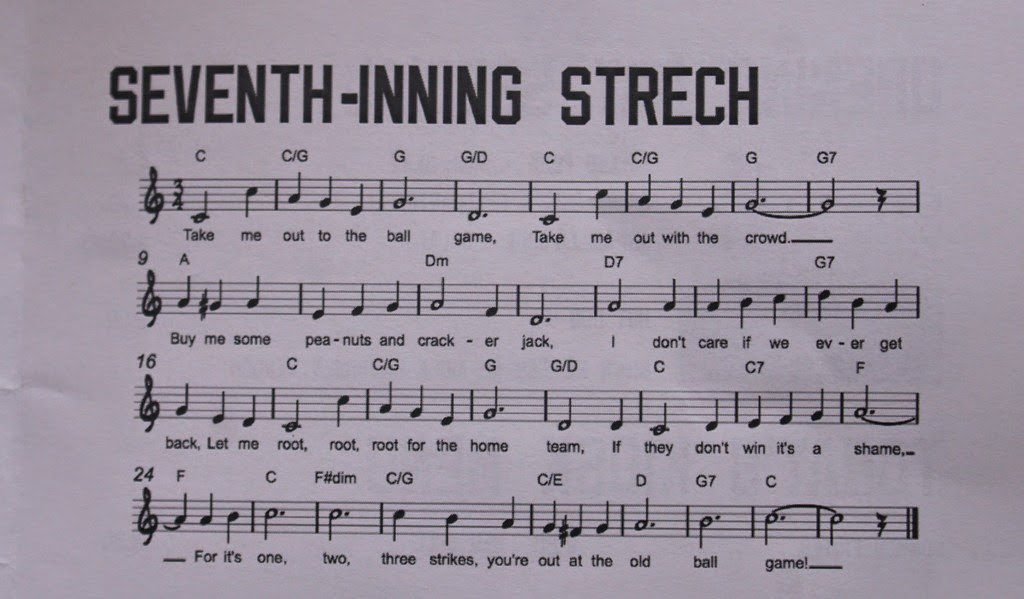The image is a horizontal, rectangular piece of sheet music displayed on a purplish-gray paper. The title at the top, written in large capital black letters, reads "Seventh Inning Stretch," though "Stretch" is misspelled. Beneath the title, the familiar baseball song "Take Me Out to the Ball Game" is notated. Each of the song's first four lines has corresponding musical notes above the lyrics, allowing musicians to play or singers to sing in key. The lyrics read: "Take me out to the ball game, take me out with the crowd. Buy me some peanuts and Cracker Jack, I don't care if we ever get back. Let me root, root, root for the home team; if they don't win, it's a shame. For it's one, two, three strikes, you're out at the old ball game!" The notation is organized neatly, with words and music clearly aligned, making it a useful tool for performing this traditional song commonly sung during the seventh inning stretch of baseball games.